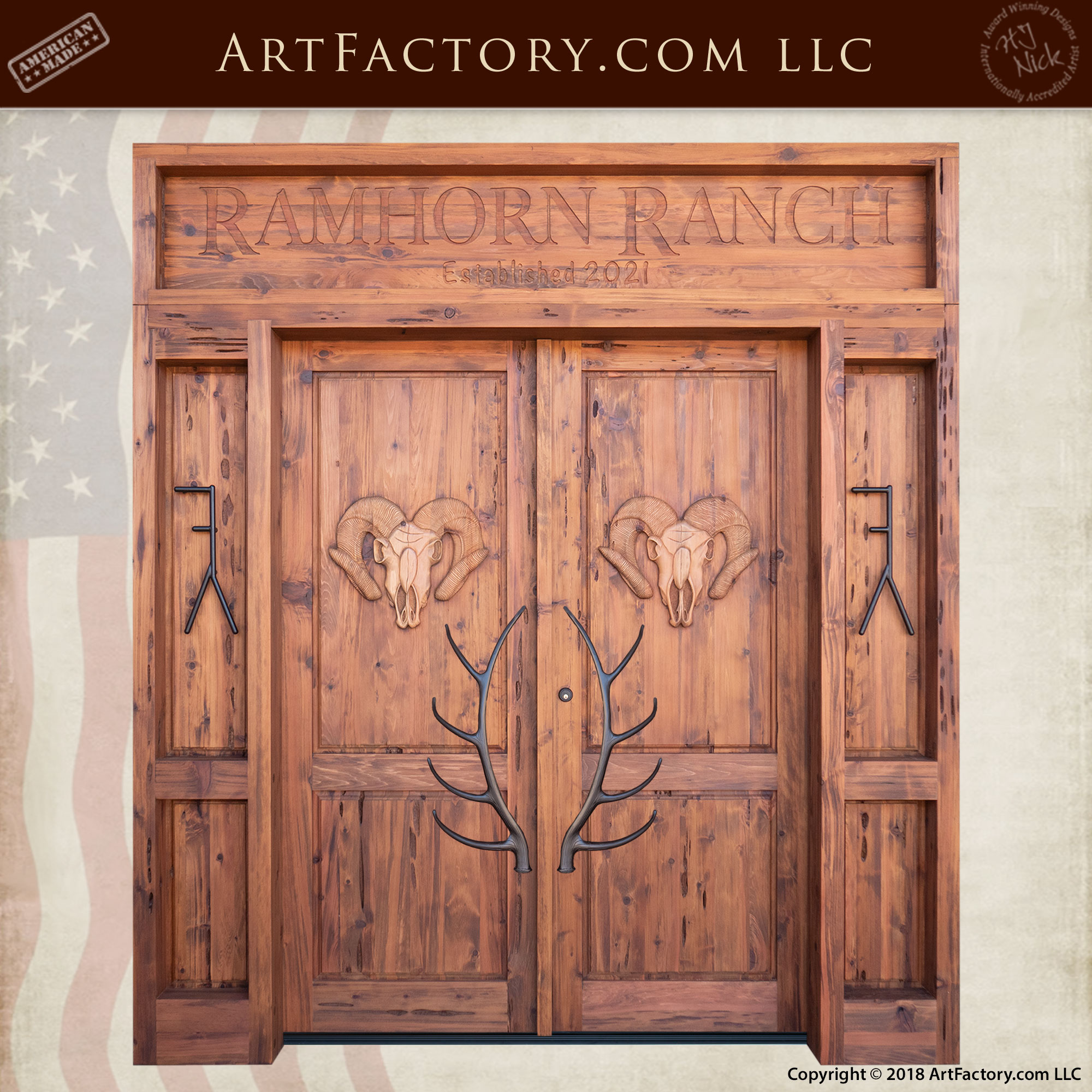The color photograph showcases an exquisite set of double wooden doors, each intricately carved with the front view of a ram, featuring long, curled horns. Above the doors, the text "Ram Horn Ranch" is artfully engraved, with "established 2021" etched in smaller letters beneath it. The door handles are strikingly fashioned to resemble black antlers, adding to the rustic charm. To the left of the door, there is a small image of the American flag, subtly placed. The background of the photograph features a grayscale, horizontally placed American flag, creating a faded yet patriotic backdrop. Additionally, over a maroon banner at the top, "Artfactory.com, LLC" is displayed, with "American Made" to the left and an emblem with "H.J. Nick" to the right, indicating the craftsmanship and origin of the doors.